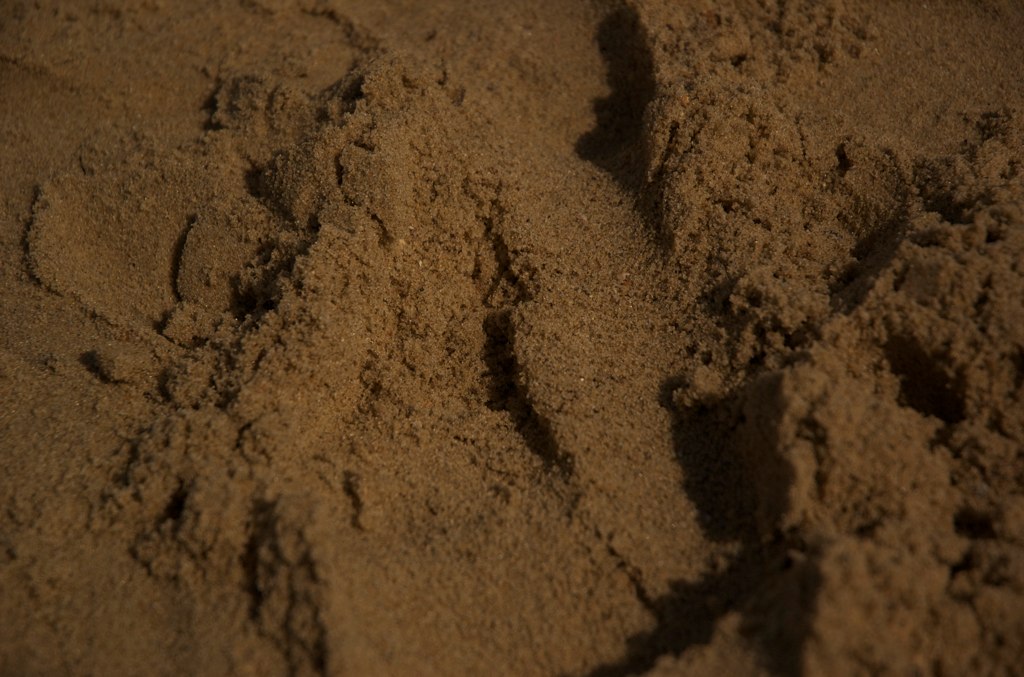This image is a highly detailed, up-close photograph showcasing a mound of moist, cinnamon brown sand or soil. The surface texture is irregular, featuring small peaks, valleys, and scoops, suggesting it has been either played with or disturbed. The lighting in the photo is dim, resulting in a slight gradient with parts appearing lighter on one side and darker on the other. The photo is taken from above, focusing solely on the sand or soil without any additional objects, text, or numbers present. The setting remains ambiguous, potentially being indoors or outdoors, such as at a beach, farmland, or a potting soil context. The fine granularity and uniform, rock-free texture dominate the entire frame.